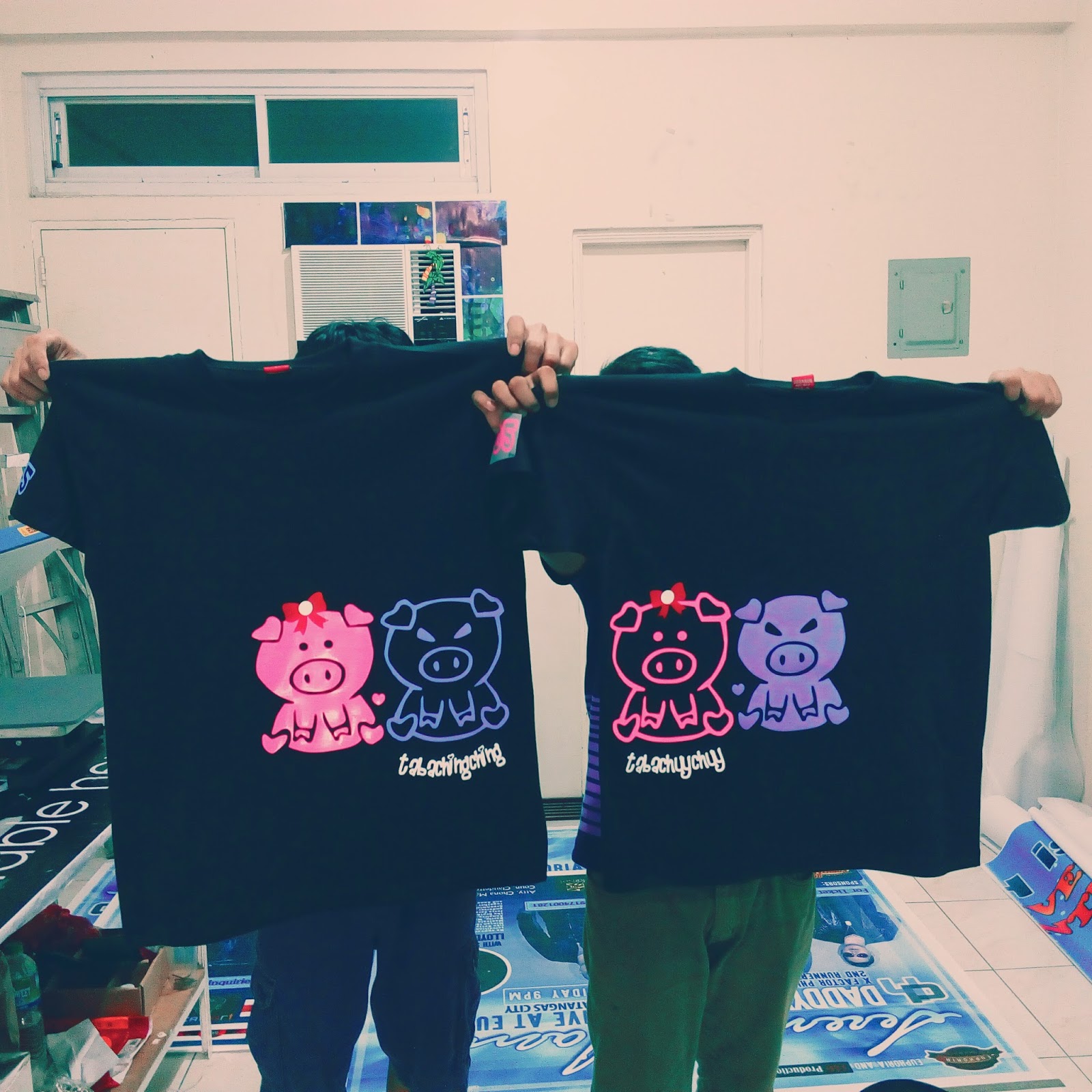In the photograph, two figures stand side by side with their faces obscured by the black t-shirts they hold up with both hands. The person on the left is wearing dark blue pants, while the person on the right is in green pants. Both figures have black hair peeking out from beneath their hats. Each t-shirt features an illustration of two pigs designed to be complementary: one shirt shows a pink pig with a red bow and a purple pig, while the other showcases a purple pig and a pink pig with a red bow. The pigs are depicted in different styles, with some appearing as solid colors and others as outlines. Below the pigs, in white cursive, are phrases that appear to be non-English; one reads "tab aching ching" and the other "tab achoo choo." These phrases may suggest a playful or thematic branding. Additionally, a poster lies upside down on the floor behind them.